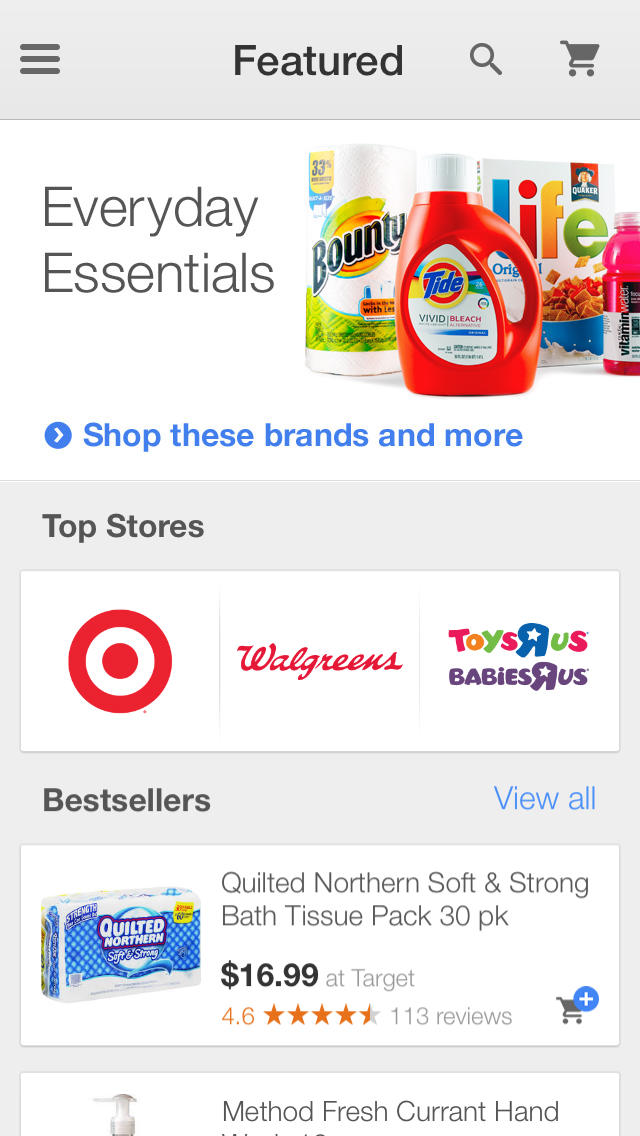This detailed caption describes a screenshot from a mobile or tablet device displaying a shopping website in portrait mode. The top of the screen features a gray navigation bar with a clickable menu icon on the left, a central search bar labeled "Glass," and a black shopping cart icon on the right. Below the navigation bar is a white banner featuring an advertisement for "Everyday Essentials," with this text prominently displayed in black font. The advertisement includes a colorful photograph depicting various household items such as cotton paper towels, Tide laundry detergent, plastic cereal containers, and a bottle of MindMine water.

Further down, the background turns gray and continues to promote "Everyday Essentials," alongside the heading "Shop These Brands and More." It showcases logos of popular stores like Target, Walgreens, Toys R Us, and Babies R Us. Beneath the heading "Top Stores," specific products are listed, such as Quilted Northern Soft and Strong toilet paper, priced at $3.35 and $6.99 at Target. Each product entry includes a thumbnail picture, customer reviews, and an "Add to Cart" button.

Finally, a partial view of another product listing is visible at the bottom of the screen, showing the top portion of a Method French Current Hand Soap box. The full details of this product are not fully visible in the screenshot.